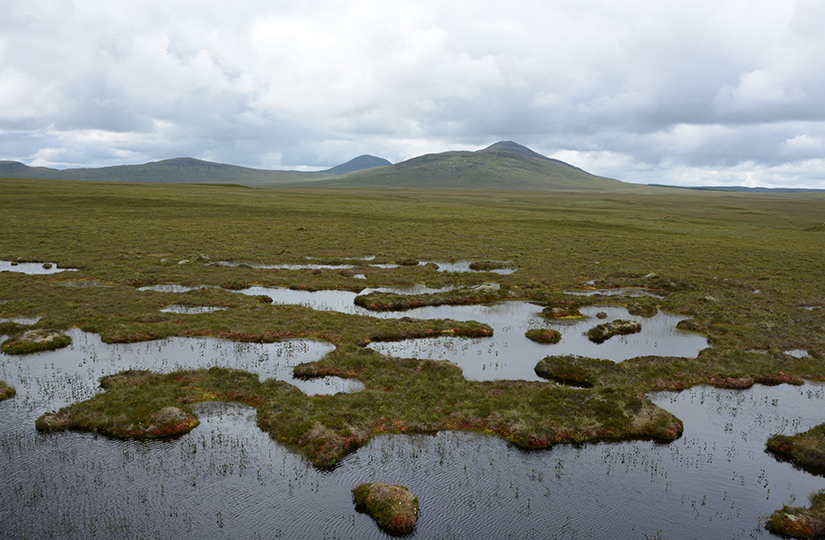This photograph captures a serene marshland landscape with a dynamic interplay between land and water. In the foreground, a watery expanse is interspersed with small islands and patches of grass, creating an intricate mosaic of wetland features. Little puddles and trails of grass weave throughout the scene, adding textures and depth. The midground transitions into bright green grassland, stretching across the image, hinting at the marsh’s verdant vitality. On the horizon, a small mountain range unfolds, characterized by two notable central peaks and tapering off into flatter terrain on the right side. The sky above is overcast with a thick blanket of gray and white clouds, enhancing the scene's tranquil yet somber mood. The overall atmosphere suggests recent rainfall, lending a fresh, albeit drab, quality to the air.